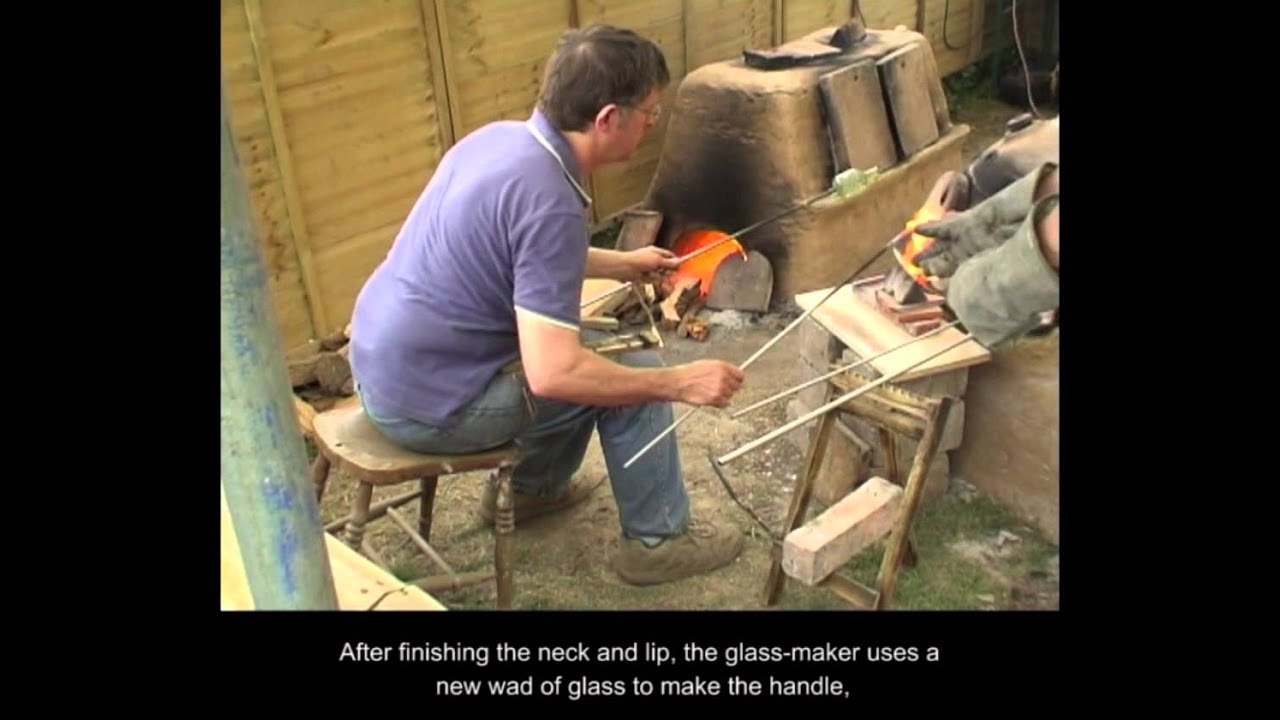In the image, a Caucasian man is seen sitting on a wooden chair without a backrest, deeply focused on the intricate process of glassmaking. He is dressed in a blue polo shirt with white trim around the collar and sleeves, complemented by worn blue jeans and well-used gray and brown shoes. The man holds two long metal rods; one of them, glowing with fiery embers, is presumably used in manipulating the glass. The other rod supports a piece of light green glass, suggesting he is in the process of crafting a vase. Behind him is a large kiln, radiating intense orange heat, hinting at the fiery temperatures within, possibly stoked by wood nearby. His hands are protected with sturdy gloves, emphasizing the dangerous yet skillful nature of his work. The scene is captioned with white text on a black border that reads, "After finishing the neck and lip, the glassmaker uses a new wad of glass to make the handle," detailing the precise stage of his craftsmanship. The colors prominent in the photo are gray, orange, blue, white, green, and black, adding to the vivid realism of this snapshot into the art of glassmaking.